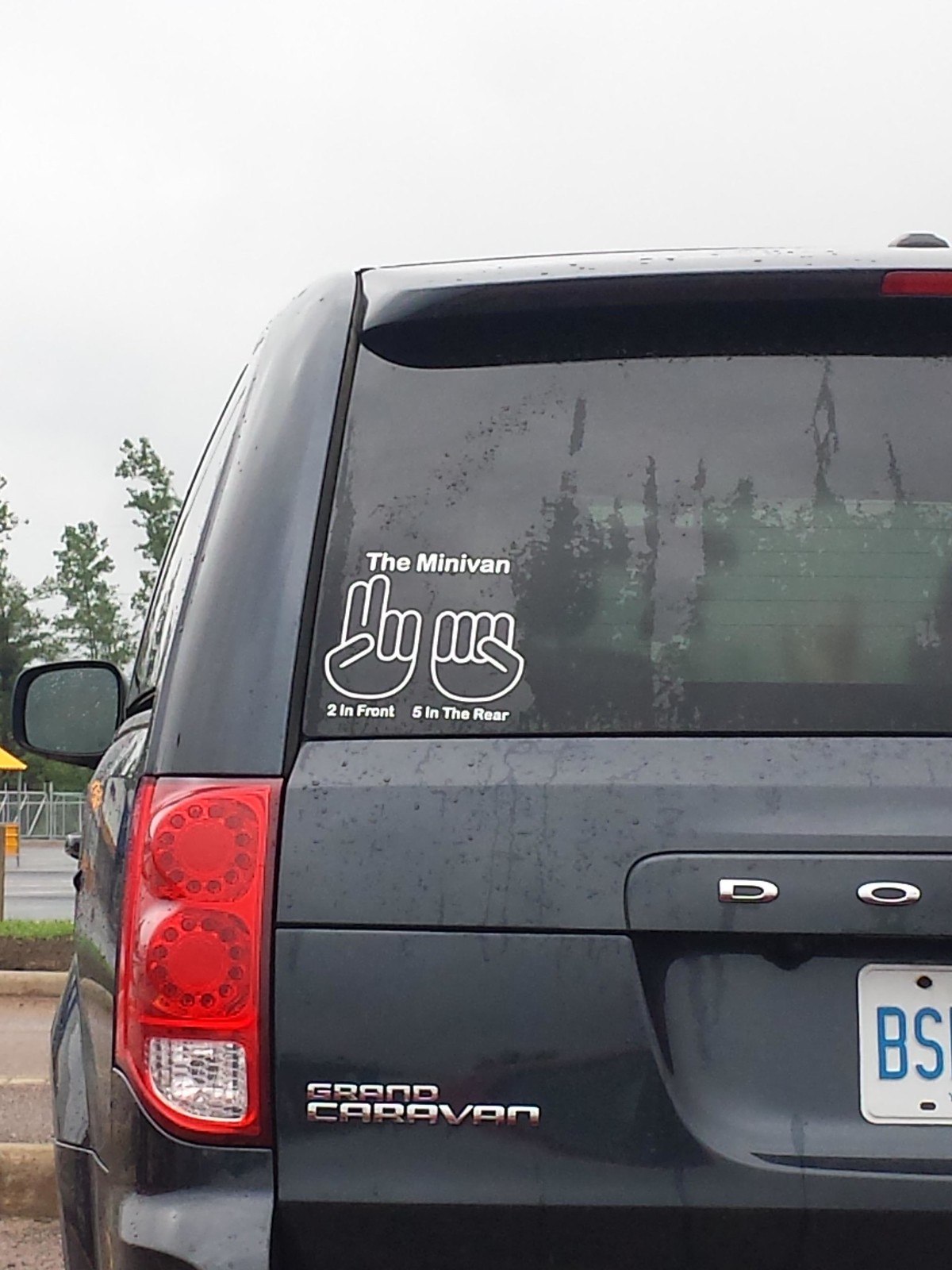This is a detailed image capturing the left half of the rear end of a dark gray Dodge Grand Caravan. On the left side, the driver's rearview mirror is visible alongside the red left taillight. The vehicle's back window features a white decal that humorously reads "The Minivan" at the top. Below this text, there are two hand signals depicted: one showing two fingers, labeled "two in front," and another showing a fist, labeled "five in the rear." A section of the license plate is visible, displaying the letters "BS" in blue on a white background. The image also hints at a cloudy day with water droplets on the vehicle, adding context to the surroundings which could be a park or a school setting.